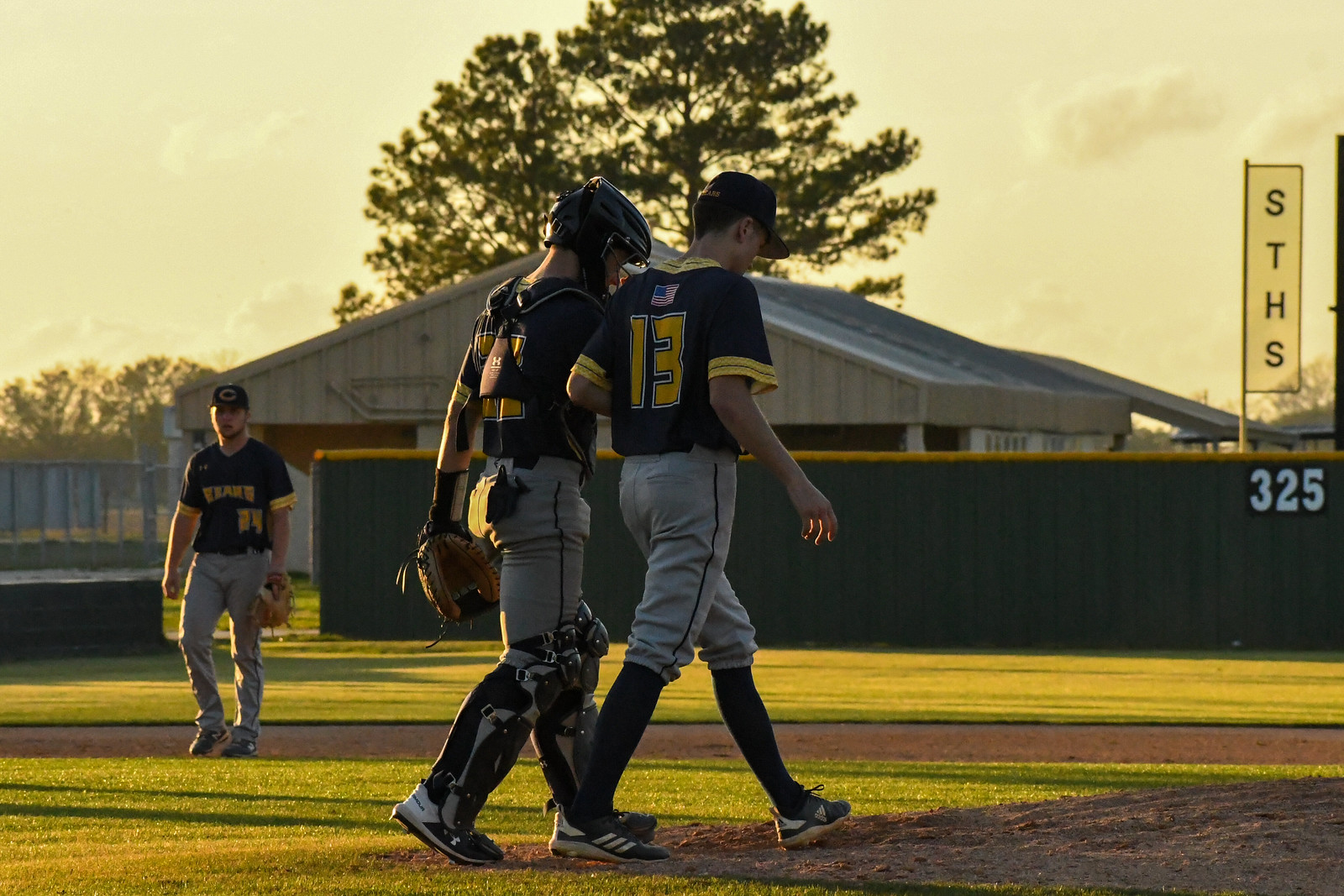The image depicts a beautifully lit baseball scene during the "magic hour" when the sun casts a golden hue over the field. This picturesque moment captures the silhouettes and details of young athletes, likely teenagers, as they transition on or off the field. In the foreground, two boys are seen walking from the left to the right. They are dressed in dark blue jerseys with gold lettering and whitish-gray pants. The boy on the right, wearing number 13, walks beside a catcher distinguishable by his helmet and leg braces, with a back harness obscuring his number. To the left in the background, another player, donning the same colors, stands with a mitt on his right hand, attentively watching his teammates. Behind them, a dark green fence with a yellow top rim stretches out, marked with the number 325 in white on the far right side. The warm, glowing light of the setting sun enhances the scene, emphasizing the dedication and camaraderie of these young athletes, beautifully captured by the photographer.